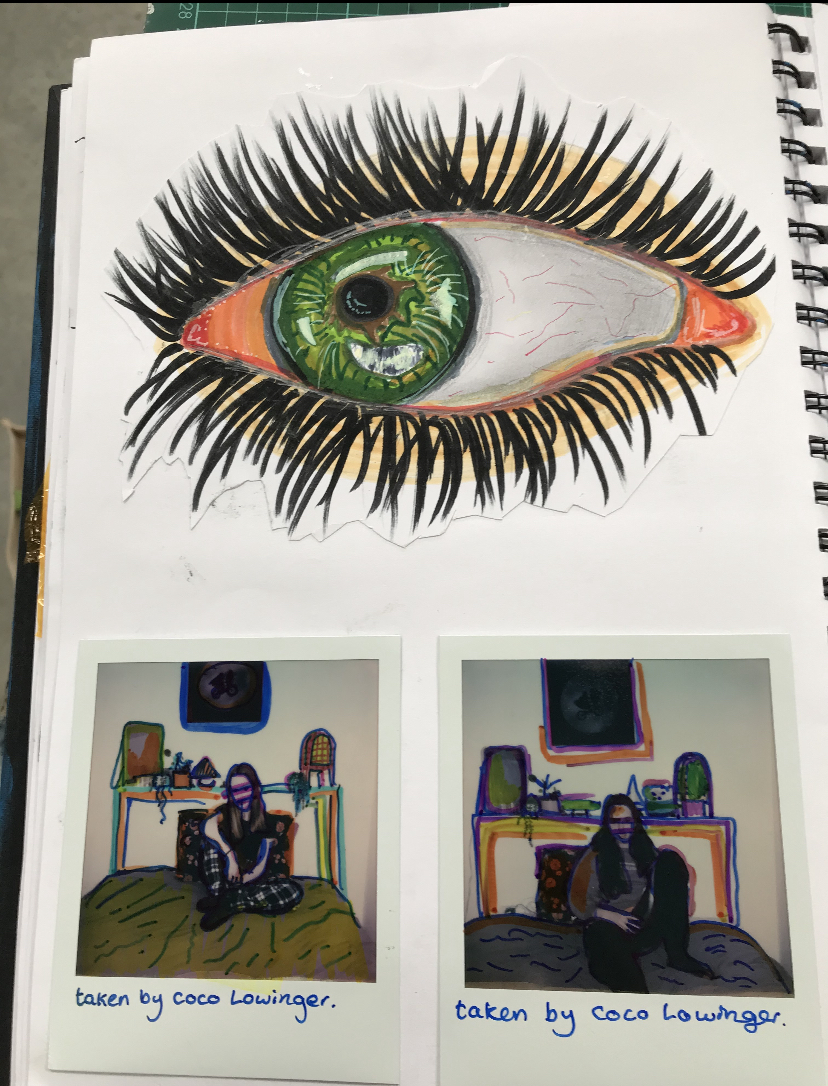The photograph captures an artist's spiral-bound sketchbook, rectangular in shape, and open to a white page towards the center, showing previous use. The coiled black wire binding is clearly visible on the right side of the page. The centerpiece of the sketch is a meticulously crafted eye with long, curled black eyelashes on both the top and bottom lids. The iris of the eye is primarily green, accented with subtle hues of blue and yellow, while the pupil is black. The whites of the eye feature fine red lines mimicking blood vessels, and the edges are tinted with a hint of red for added realism. The entire eyepiece appears to have been cut from another sheet and carefully glued or taped onto the sketchbook page.

Beneath the eye, two Polaroid photographs are affixed. These photos ostensibly depict individuals in a bedroom setting. The left image shows a girl seated on a bed, adorned with a headboard decorated with various colored items, possibly colored in by hand. The scene also includes plants, a mirror, and other decorative objects, along with a distinctive image of a boy on a bicycle with E.T. in the basket flying against a backdrop of the moon. The right image likely portrays a male figure. Both Polaroids have been personalized with color pens, adding vibrant details to the originally black-and-white prints. Each photograph is annotated with the handwritten note "taken by Coco Lowinger" in blue ink on the white borders of the Polaroids.